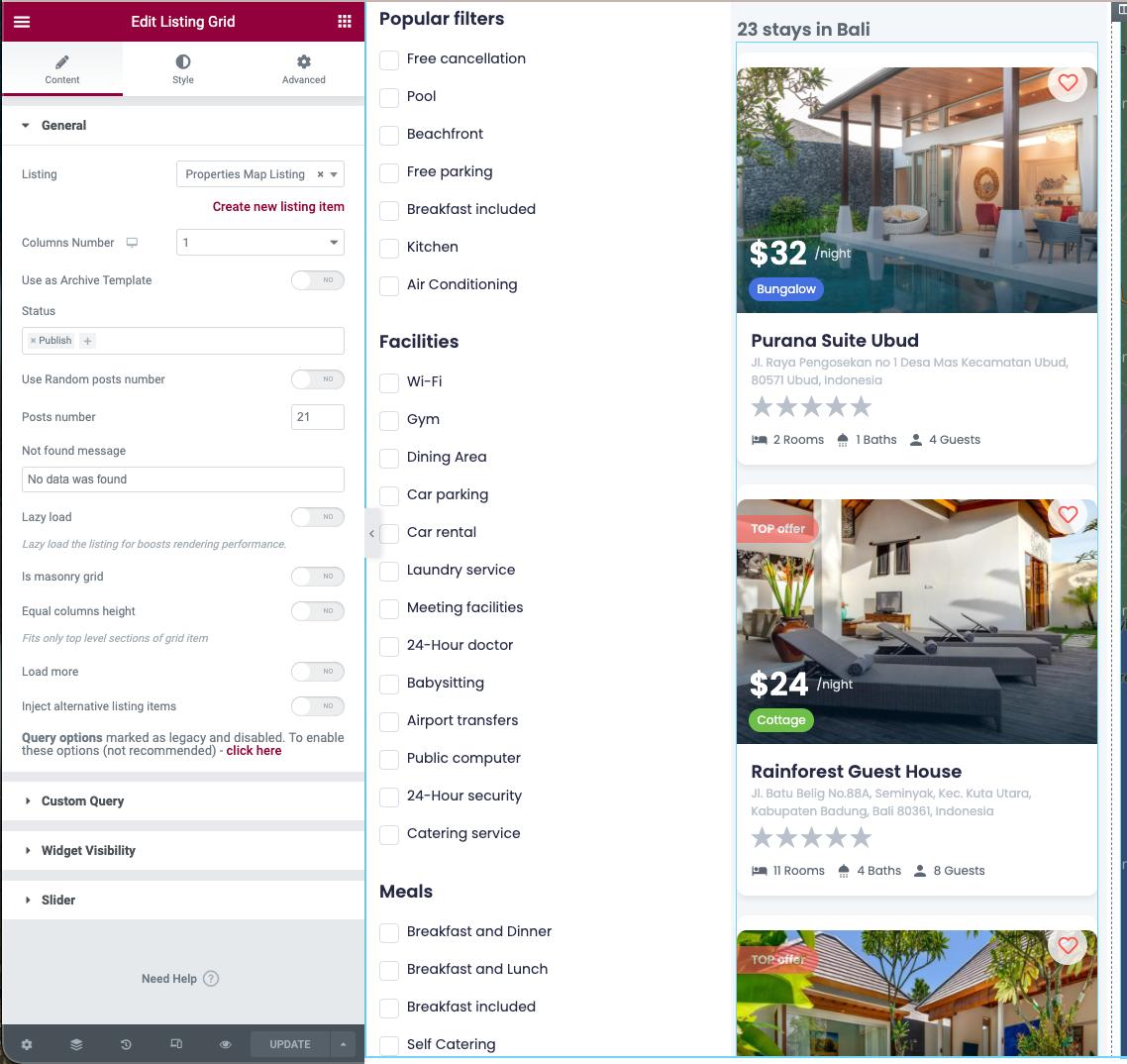The image depicts the interface of a real estate website, specifically focused on editing a listing grid. The page appears to be a comprehensive tool for managing rental property listings. 

At the top, the header is titled "Edit Listing Grid," indicating functions available for customizing how property listings are displayed. The options here include "Content," "Style," and "Advanced" settings, with "General" highlighted in bold black text. Available attributes in this section are "Listing Columns Number," "Uses," "Active Template," and "Status." Further down, options expand to "Post Number," "Lazy Load," "Masonry Grid," "Load More," "Custom Query," "Widget Visibility," and "Slider" — all prominently marked in dark black for emphasis.

On the right side of the interface, there is a section called "Popular Filters," detailing several filtering options such as "Free Cancellation," "Pool," "Beachfront," "Free Parking," "Breakfast Included," "Kitchen," and "Air Conditioning." Additional facilities that can be filtered include "Wi-Fi," "Gym," "Dining Area," "Car Parking," "Car Rental," "Laundry Service," "Meeting Facilities," "24-Hour Doctor," "Babysitting," "Airport Transfers," "Public Computer," "24-Hour Security," and "Catering Service." 

Under the meals category, there are various options listed: "Breakfast and Dinner," "Breakfast and Lunch," "Breakfast Included," and "Self-Catering."

The image also provides a glimpse of three types of rental places. The first is priced at $32 per night. The second, described as a cottage, costs $24 per night. The third option is marked as a "Top Offer," but the price is cut off at the bottom of the image, making it unreadable. 

A gray-shaded prompt is visible within the interface stating “Need help?” followed by a question mark, likely linking to customer support or a help section.